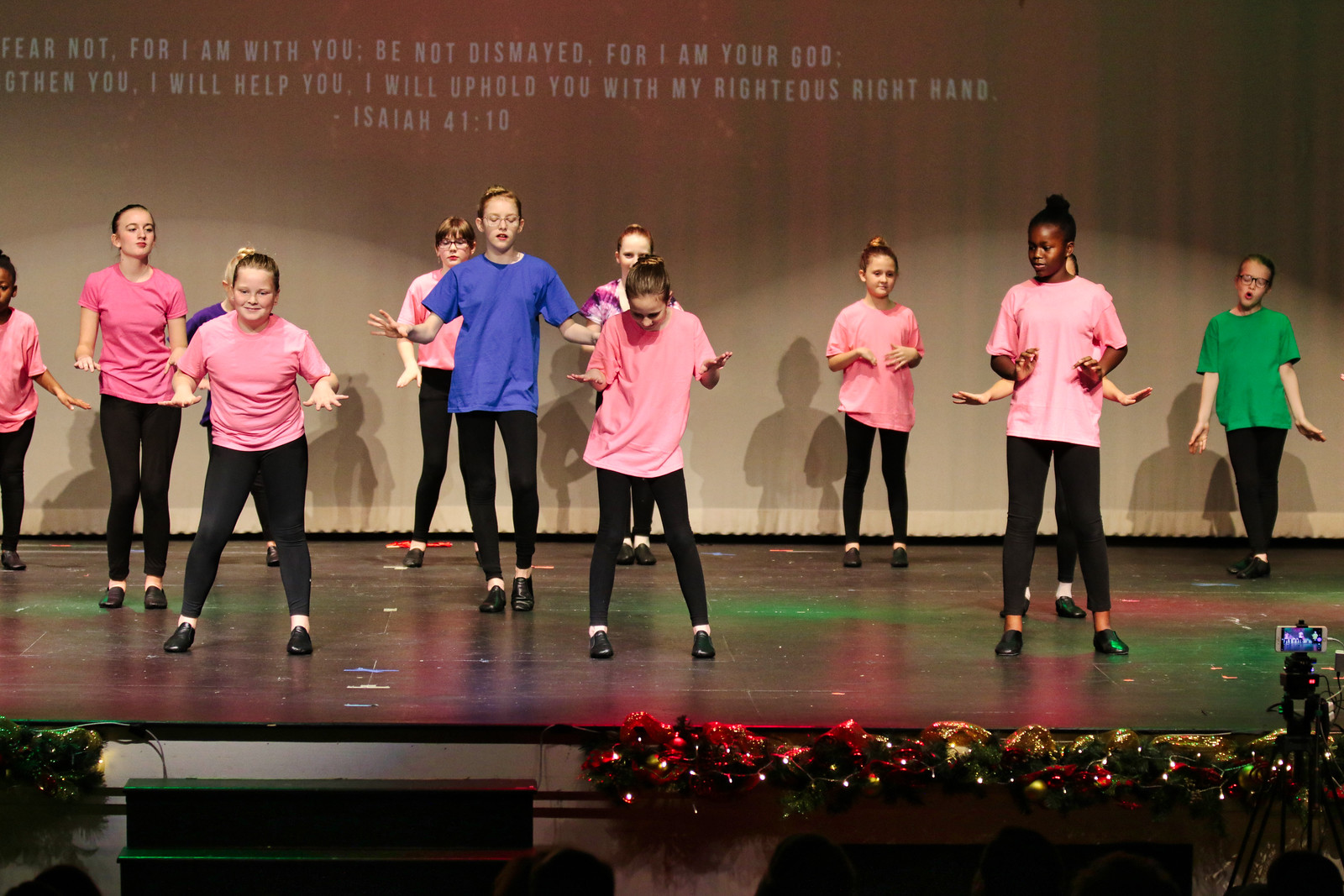The full-color photograph captures a lively Christmas dance recital set on an indoor auditorium stage featuring a group of prepubescent children, approximately 10-11 years old. The majority of the children, primarily girls, are dressed in pink tops paired with black leggings and black shoes. Among them, a few girls stand out in different colored tops—a blue t-shirt in the middle, a green t-shirt on the far right, and a pink tie-dye top in the back corner. Two boys also participate, one in a blue shirt and another in a green shirt. Christmas decorations adorn the bottom of the stage, adding to the festive atmosphere, and a camera on a tripod is set up to record the event. The backdrop features a white curtain with a projected Bible verse, Isaiah 41:10, which reads, "Fear not, for I am with you. Be not dismayed, for I am your God. I will help you, I will uphold you with my righteous right hand."